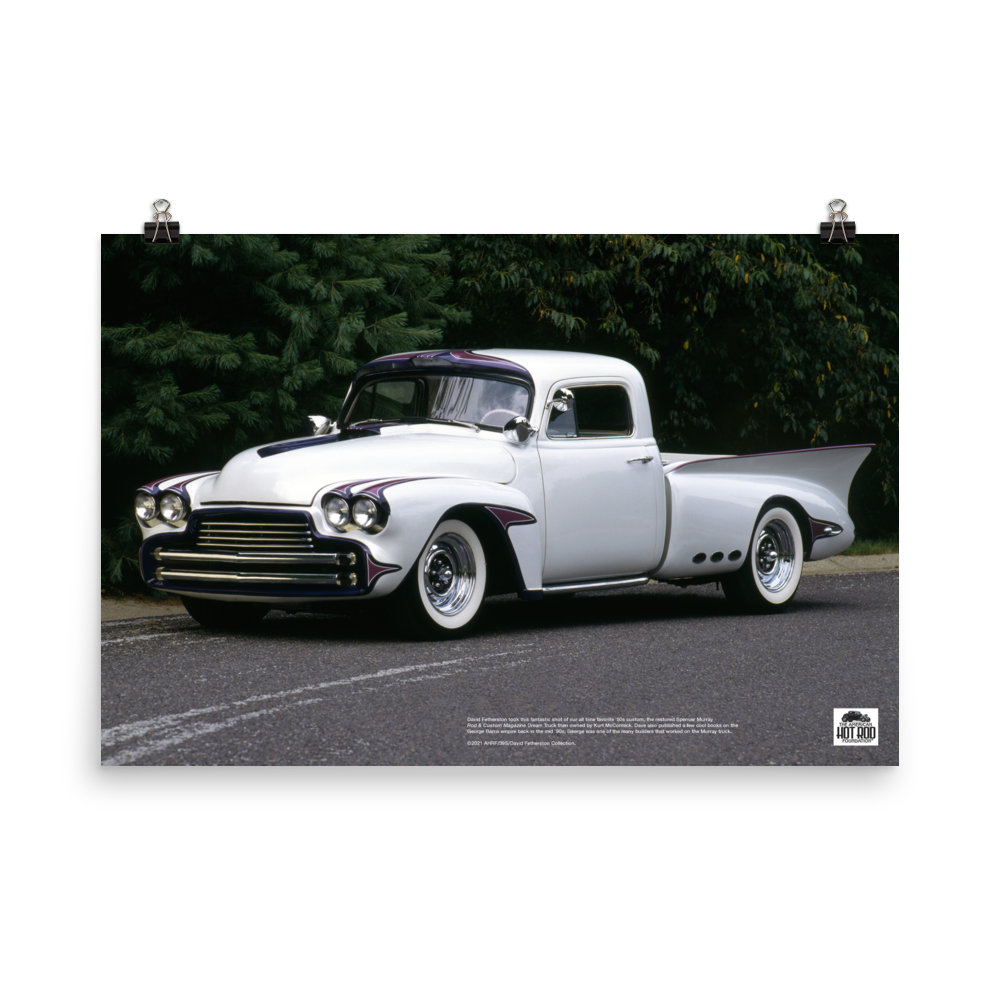The image showcases a meticulously modified vintage truck, prominently featured against a white wall, secured by two clips. The truck, predominantly white with black and purple accents, exudes a classic yet custom allure reminiscent of a car magazine spread. Its front end boasts four headlights and a two-piece chrome bumper beneath, accompanied by a black hood section. Enhancing its unique aesthetic, the roof near the windshield displays a striking design in blue, purple, and red, resembling wings. The open truck bed at the rear is accentuated by grand fins evocative of late 50s and early 60s Cadillacs. The vehicle is set against a backdrop characteristic of an asphalt road flanked by dense bushes, with white-wall tires completing its vintage look. Notably, the absence of an outside mirror hints at the truck's age and vintage appeal. In the bottom right-hand corner, "Hot Rod Magazine" is prominently displayed, emphasizing the truck's standout recognition.